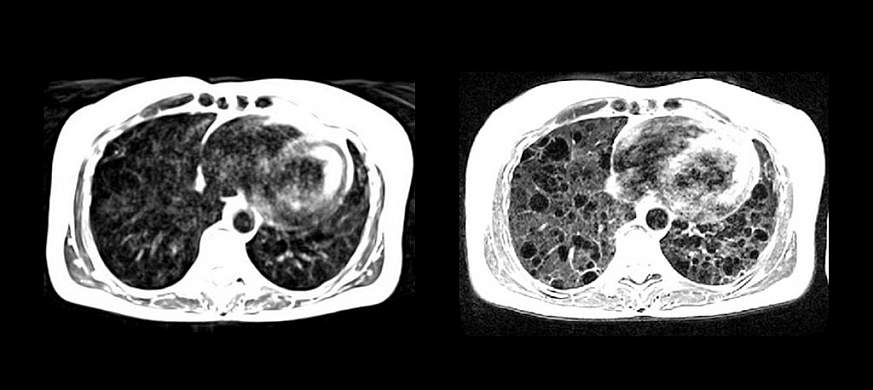This image displays two side-by-side x-rays of a pelvis, set against a black background, creating a landscape orientation. The white, slightly curvy, rectangular outlines of the pelvises stand in stark contrast to the dark background. The left x-ray has a darker, fuzzier interior with two kidney-bean or drop-shaped areas, while the right x-ray appears lighter and more detailed. It reveals smaller, clear, round black circles within its gray interior. Both x-ray sections have distinctive bulbous forms located at the top right center. The image is notably wider than it is tall, reinforcing the landscape presentation and the division into two distinct, yet similar halves.